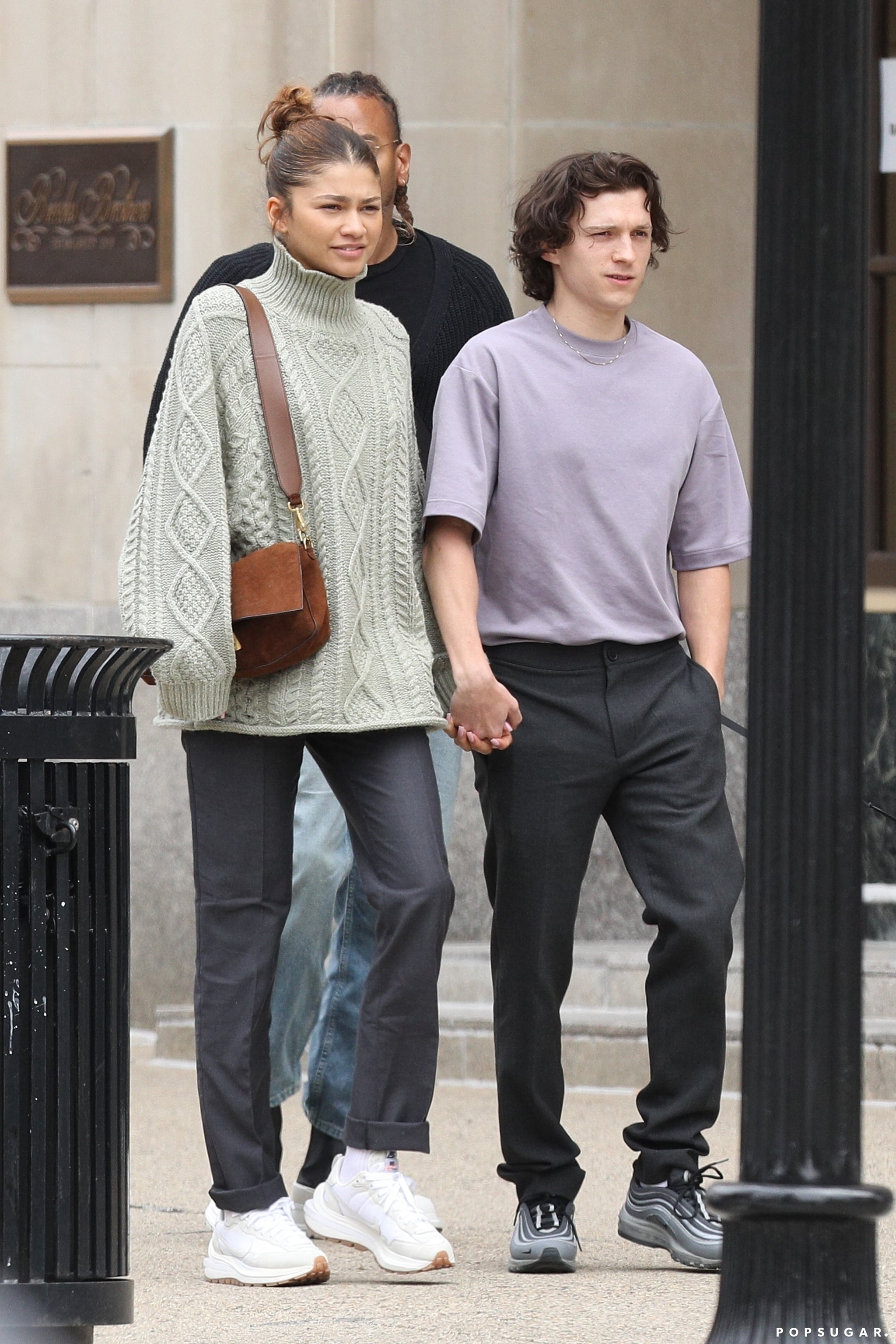In this candid paparazzi photo taken outside on a sidewalk in what appears to be a larger city, Zendaya and Tom Holland are seen walking hand in hand. Zendaya, who has light brown skin and dark brown hair styled in a messy bun, is wearing an oversized off-white turtleneck sweater with long sleeves that cover her hands, dark gray pants rolled at the cuffs, and white sneakers. She accessorizes with a small brown purse slung over her right shoulder. Tom Holland, standing to her right, has light skin and wavy, slightly longer dark hair. He is dressed casually in a light lavender t-shirt, black pants, gray sneakers, and a small silver chain necklace. His right hand holds Zendaya's left, and his left hand is tucked into his pocket. Behind them, partially obscured by Zendaya, is a larger black man with braided hair who appears to be their bodyguard. He is wearing a black sweater and blue jeans. The setting includes a black street lamp pole on the right side of the image and a black metal trash can on the left. The bottom of the image features the text "Pop Sugar."